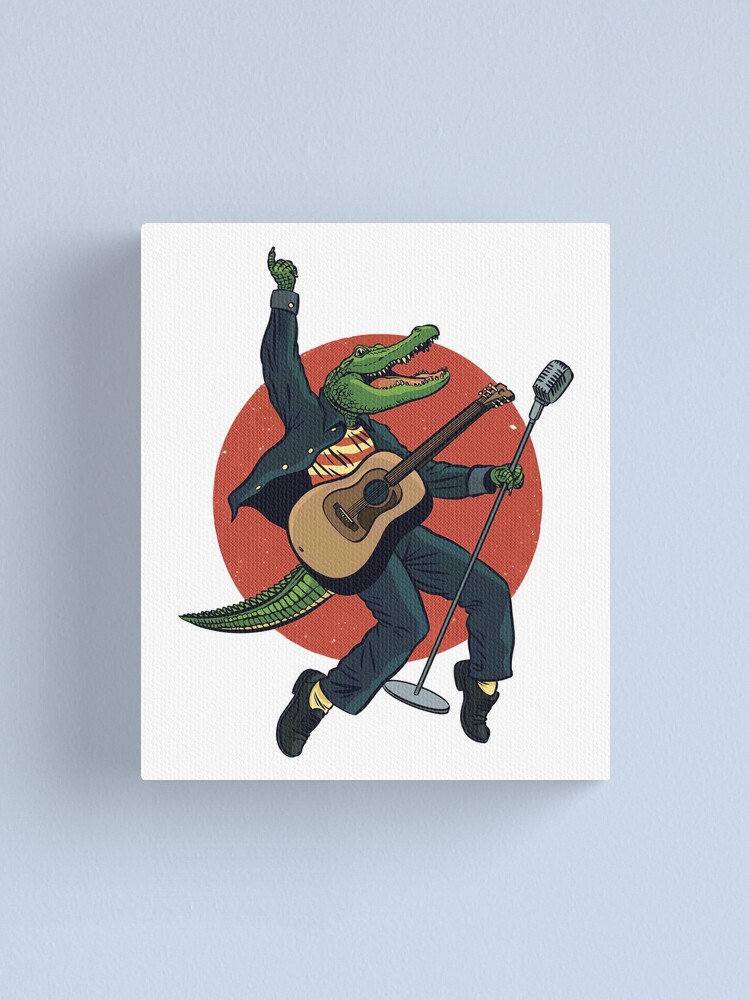This colorful artwork displays a white canvas positioned centrally on a light blue or gray background. At the heart of the composition is a large, solid red circle. Positioned dynamically in front of this circle is an anthropomorphized alligator, striking a pose reminiscent of iconic performers like Elvis Presley and Michael Jackson. The alligator's figure is expressive, with knees bent and standing on the tips of its toes, exuding an energetic, performance-ready stance.

The alligator's left hand firmly grips a microphone stand, which it tips slightly forward, while its right hand is raised, pointing upwards with an outstretched finger. Its mouth is wide open, showcasing sharp teeth, as if passionately singing into the microphone. The alligator dons a stylish outfit: a denim jacket layered over a red and white striped shirt, paired with tight blue pants, white socks, and black dress shoes or loafers. An acoustic guitar is strapped across its waist, though it isn't being played in the moment depicted.

The vivid combination of colors—the blue backdrop, the white canvas, and the prominent red circle—enhances the theatrical and surreal nature of the scene. The artwork captures a vibrant, dynamic moment, marrying elements of music, performance, and fantasy through its unique central figure.